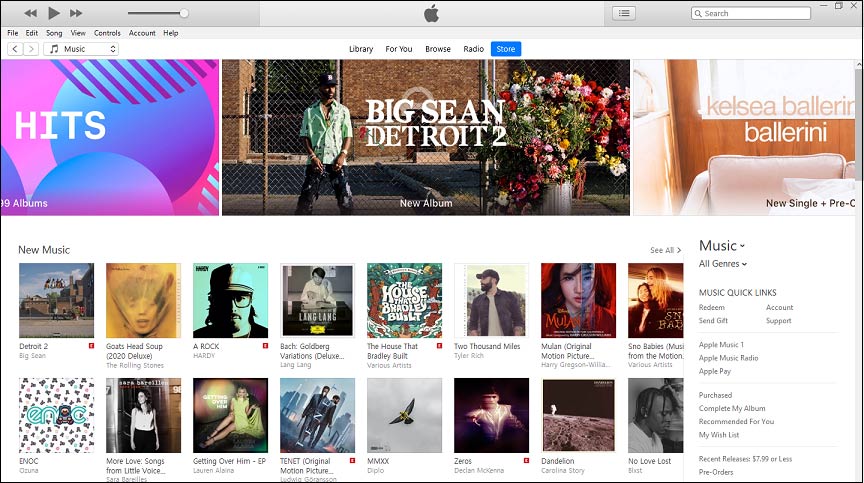The image is a screenshot from Apple Music, showcasing its interface. At the top center, an Apple logo is prominently displayed. To the top left, navigation controls are visible, including 'Back', 'Play', 'Forward', and a volume slider. The top right features a search bar. Below the top navigation, there is a menu bar with options: File, Edit, Song, View, Controls, Account, Help.

Beneath the menu bar, there is a section highlighting various categories: Library, For You, Browse, Radio, Store. The 'Store' category is selected, indicating the current view. 

This view displays featured content at the top, including segmented tabs like 'Hits', 'Big Sean - Detroit 2 (New Album)', and 'Kelsea Ballerini - New Single'. Below these tabs, several music thumbnails are arranged, showcasing new releases such as 'Detroit 2', 'A-Rock', 'A House That Bradley Built', and '2,000 Miles'.

Additionally, there is a detailed dropdown menu emerging from the bottom right corner, listing options like Music, All Genres, Music Quick Links, Redeem, Send Gift, Account Support, Apple Music, Apple Music Radio, Apple Pay, Purchase, Complete My Album, Recommended For You, My Wishlist, Recent Royalties, $7.99 or less, and Pre-Orders. The dropdown consolidates various purchasing and account support options within the Apple Music ecosystem.